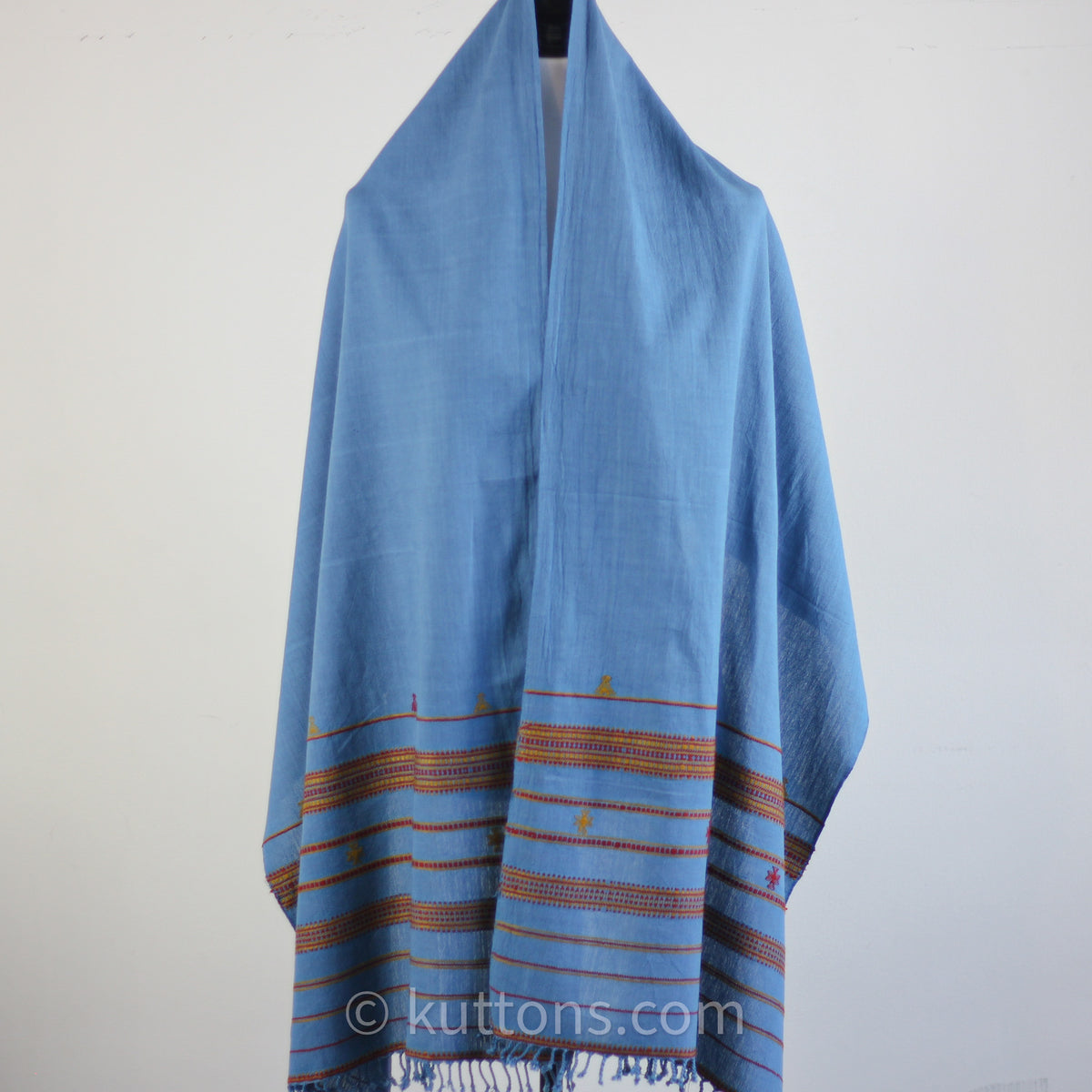This image features a wide vertical shawl draped over a mannequin, which is visible from the neck down to around mid-thigh or knee length. The background is a very light gray, creating a neutral contrast to highlight the shawl. The material of the shawl is predominantly light blue and it appears to be wide, almost like a large scarf. The upper portion of the shawl is plain blue, while the lower half is adorned with intricate embroidery in horizontal lines of dark brown, light brown, and possibly dark reddish-brown threads. Additionally, there are gold, purple, and orange embroidered details, along with a notable gold cross design. Toward the bottom, the shawl features light blue tassels that hang down. On one side, at the bottom, there is a circle with the letter "C" for copyright followed by the text "Kuttons.com K-U-T-T-O-N-S". The shawl is slightly gathered in the front, emphasizing its luxurious drape over the mannequin, whose head is not visible in the image.